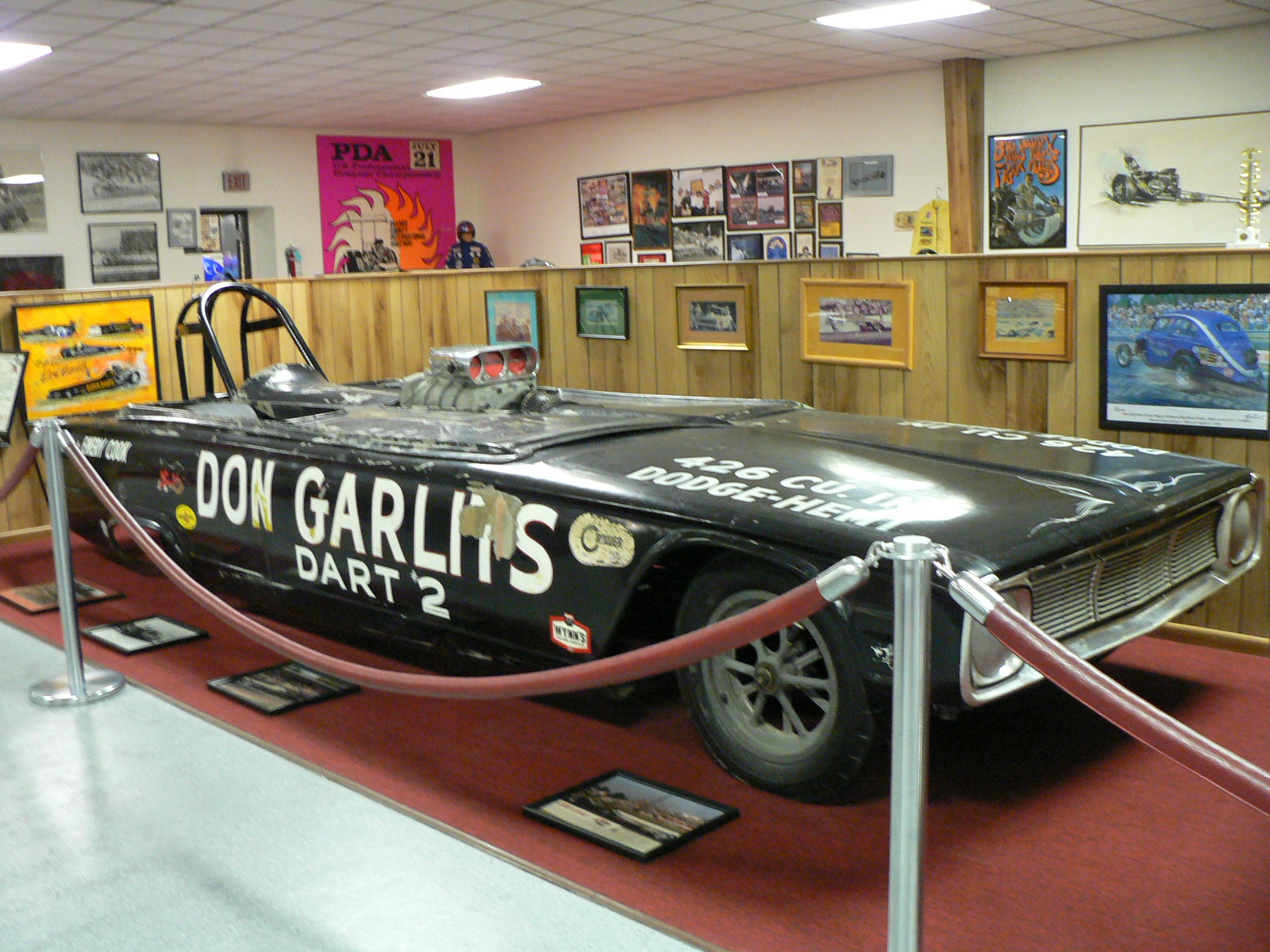In the image, a vintage drag racing car, identified as Don Garlits' Dart 2, takes center stage, set diagonally on a pink carpet within a showroom or museum setting. The car, an elongated and futuristic-looking black design, features distinctive text indicating its specifications: "Don Garlits Dart 2," "426 CU," and "Dodge Hemi," though some details are partially obscured by glare. A unique feature of the vehicle is a rocket-like engine protruding from its midsection, adding to its sci-fi aesthetic, and it appears to be a single-seater with a U-shaped metallic structure possibly outlining the cockpit area.

Surrounding the car, there are numerous visual elements enhancing its display. Directly behind it stands a substantial wooden wall adorned with various posters and photographs, establishing a nostalgic atmosphere. The scene is framed with red barriers that restrict close access. The back third of the image showcases more posters on a white wall, beneath a ceiling equipped with fluorescent lights. The overall setting, rich in varied colors – blacks, whites, reds, grays, yellows, pinks, oranges, and blues – reinforces the nostalgic yet futuristic aura of this unique exhibit.